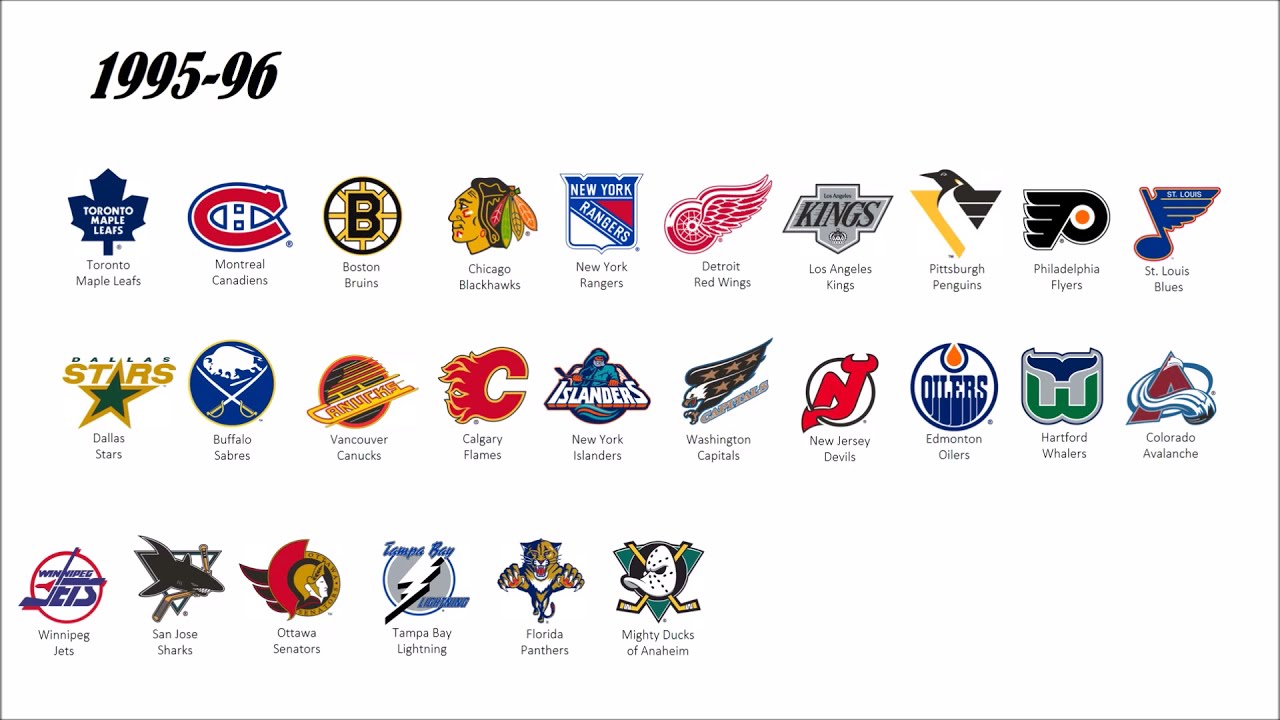The image is a promotional poster for hockey teams from the 1995-1996 season, set against a white background. At the top of the poster, the text "1995-1996" is displayed prominently in black font. The poster features the logos and names of numerous hockey teams, arranged in rows. The teams include the Toronto Maple Leafs, Montreal Canadiens, Boston Bruins, Chicago Blackhawks, New York Rangers, Detroit Red Wings, Los Angeles Kings, Pittsburgh Penguins, Philadelphia Flyers, St. Louis Blues, Dallas Stars, Buffalo Sabres, Vancouver Canucks, Calgary Flames, New York Islanders, Washington Capitals, New Jersey Devils, Edmonton Oilers, Hartford Whalers, Colorado Avalanche, Winnipeg Jets, San Jose Sharks, Ottawa Senators, Tampa Bay Lightning, Florida Panthers, and Mighty Ducks of Anaheim. The logos are neatly arranged, capturing the essence of the hockey league from that specific season.